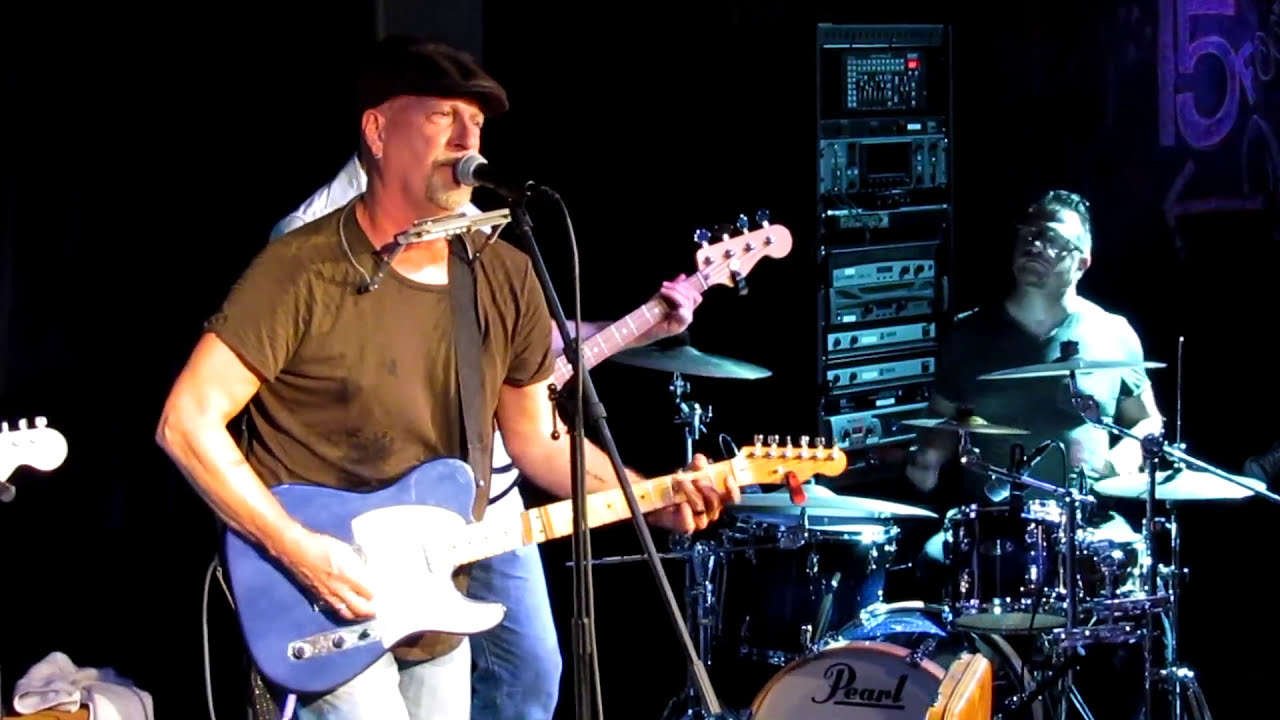The image is of a live concert performance set against a black background, with focal emphasis on an older white man who occupies the forefront. He sports a black beret, olive green shirt, and blue jeans. With a gray goatee and mustache, he stands center-left, gripping a blue Fender guitar with a white pickguard and light wood neck. A strap runs over his shoulder, and he has a harmonica encased in a holder around his neck as he sings into a microphone on a stand. To the left of the main performer (stage right), a portion of another guitar and the hand of a bass player can be seen, though the player’s face is obscured. On the far right is a drummer, partially illuminated with aqua lighting, seated at a black Pearl drum set with cymbals. The background features extensive recording equipment in a server-rack arrangement. In the upper right corner of the image, there is the number "15" with an arrow beneath it, seemingly drawn in chalk.